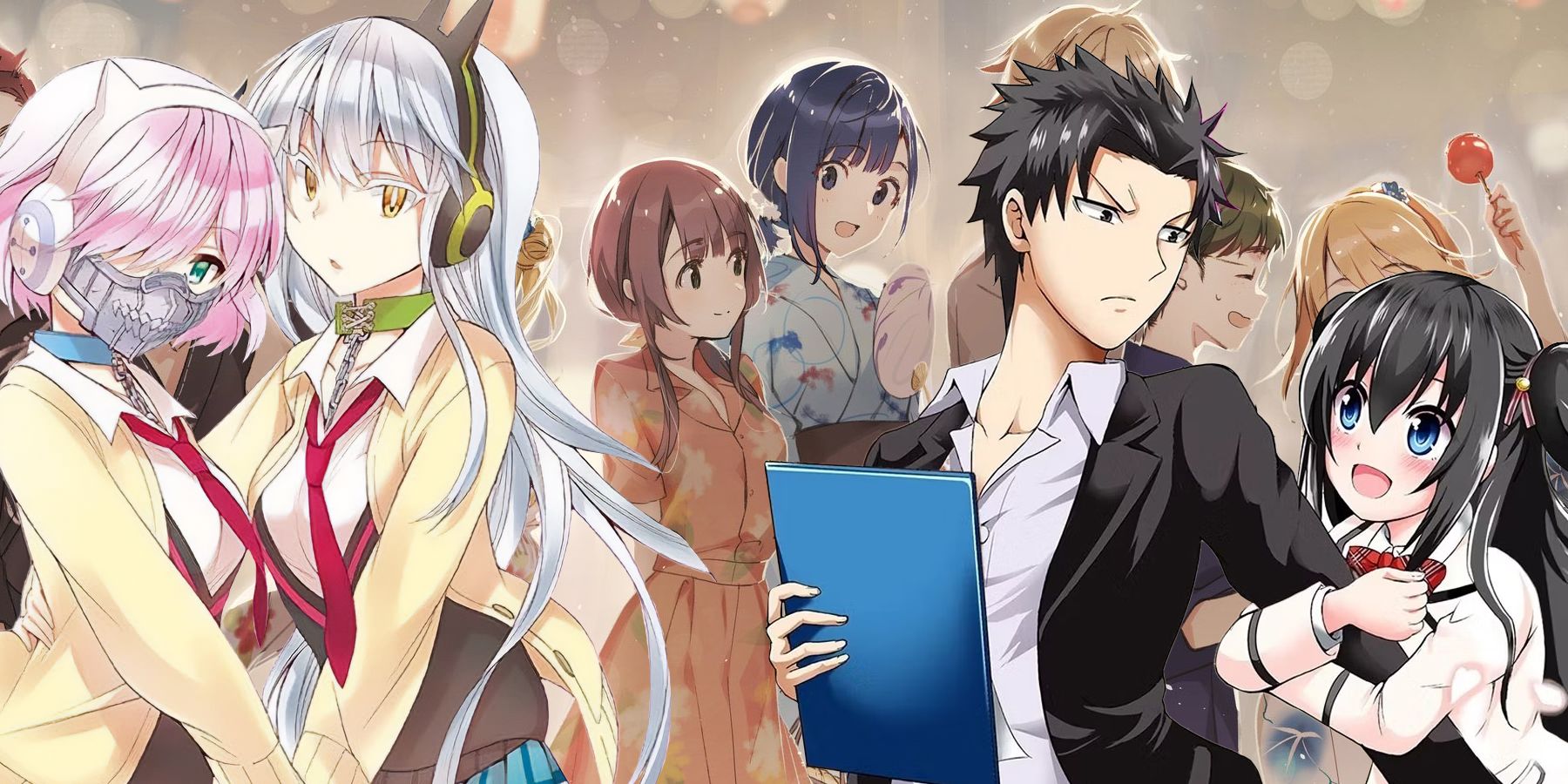The image presents a diverse array of anime characters, each rendered in unique yet distinctly Japanese anime styles. On the far left, there are two schoolgirls adorned with cat ear headphones and collars with chains. The leftmost girl, with pink hair and cat ear headphones, wears a face mask decorated with a toothy design, while the girl beside her has long white hair, yellow eyes, and black cat ear headphones. Next to them, at the center of the image, stands a young man in a black suit jacket and white button-down shirt, holding a blue tablet. Clinging to his left arm is a small girl with big blue eyes and long black hair, dressed in a school uniform. Behind these central figures, more muted anime girls in traditional kimonos populate the background, adding a serene contrast to the vibrant foreground characters. The scene is a vivid collage, capturing the essence of various anime themes and character designs, enriched by an array of colors including blues, pinks, grays, pale yellows, lime greens, oranges, blondes, blacks, beiges, tans, and whites.